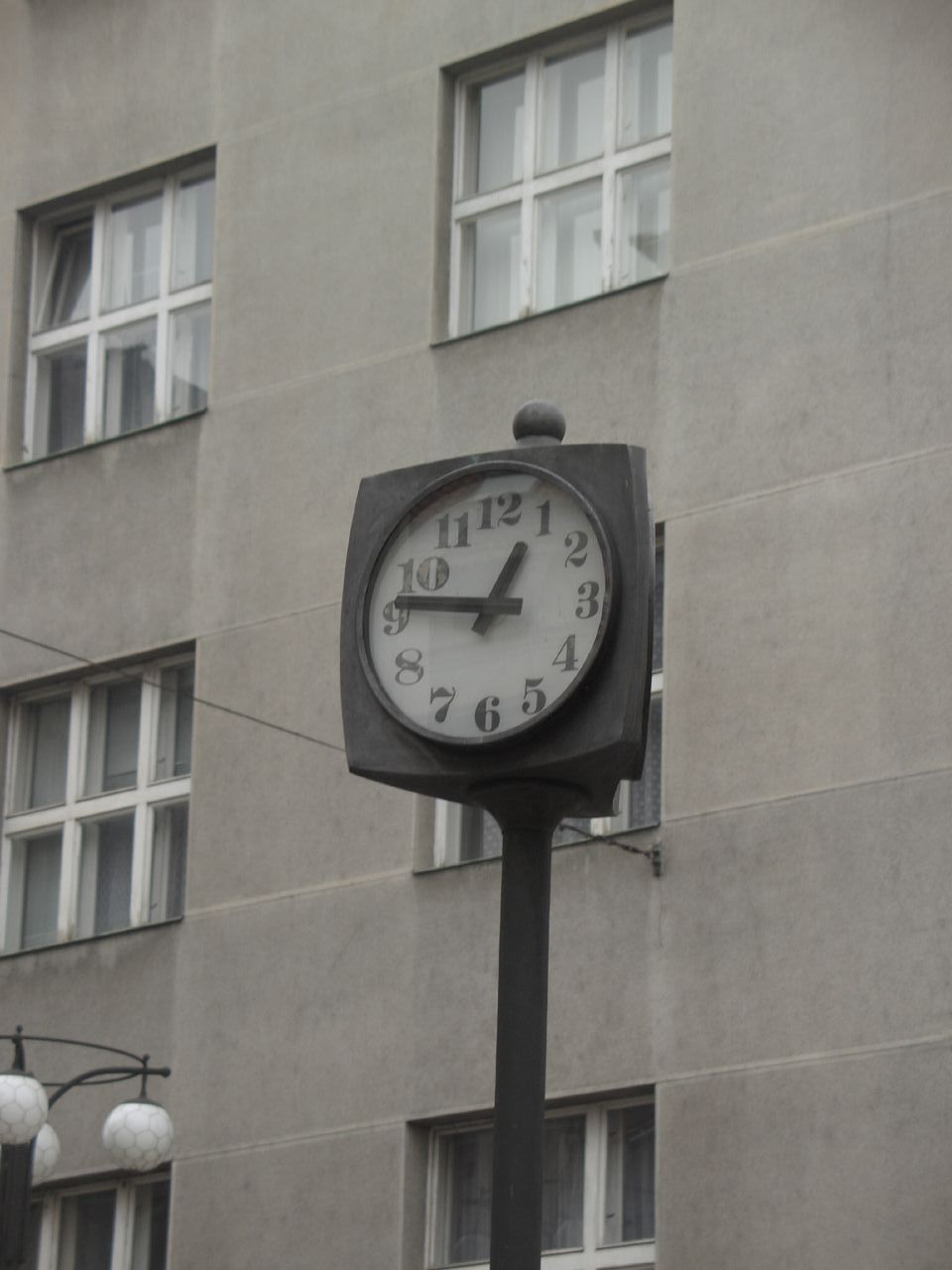A striking image captures a tri-sided clock, prominently displayed on a post in front of a stately gray building. The clock, designed to be visible from any direction, features elegant, flourished numerals with large serifs, adding a touch of sophistication to its appearance. The time displayed is a quarter to one in the afternoon, as evidenced by the daylight ambiance in the scene. The building behind the clock is constructed from either stone or concrete, and its façade includes six windows, each framed in pristine white paint. The clock itself, with a dark brown exterior, stands in contrast to the lighter tones of the building, making it a focal point of the image.